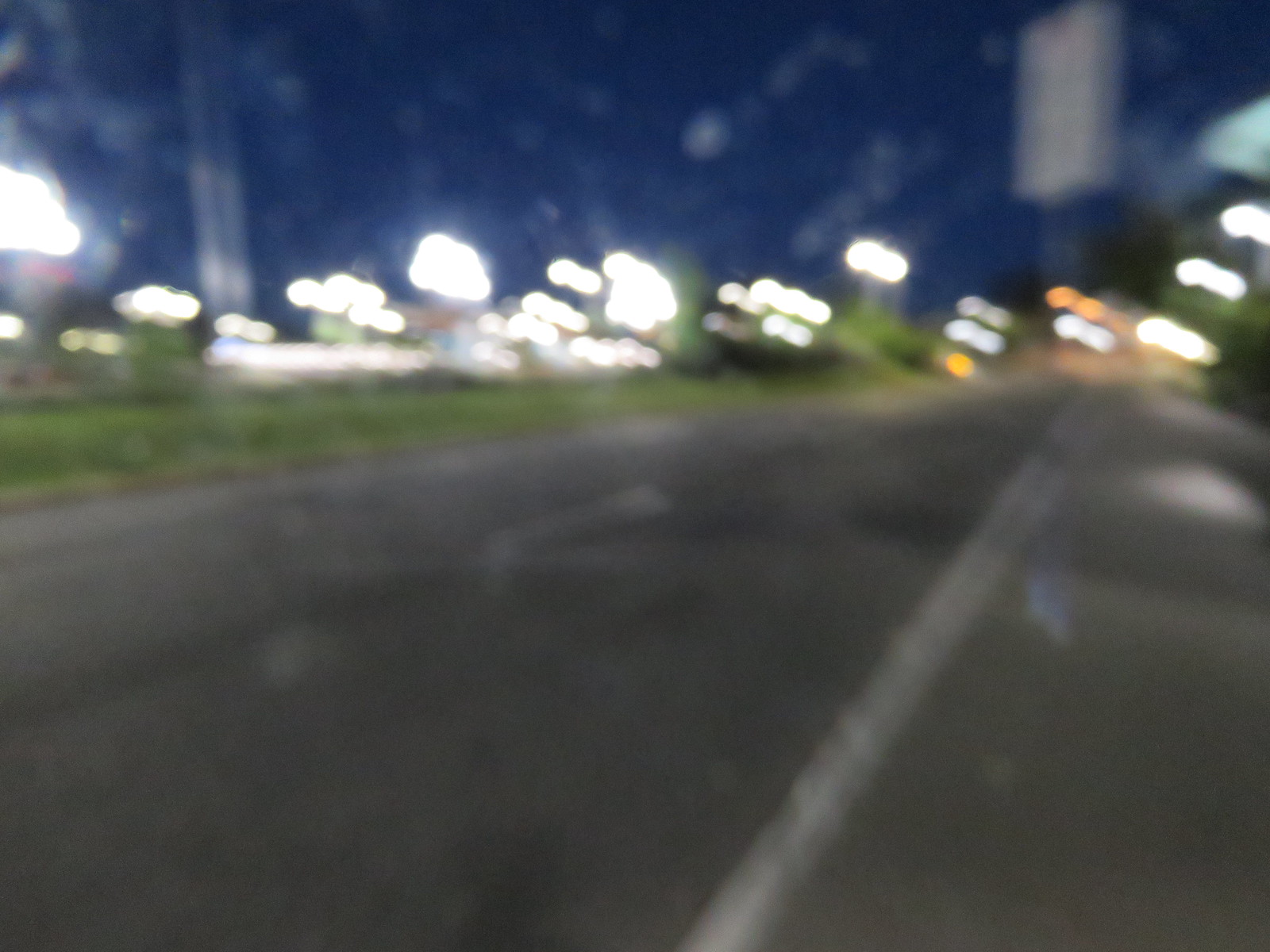A blurry street scene captures an urban landscape shrouded in motion or out-of-focus distortion. The pavement in the foreground is slightly discernible, hinting at a typical street surface. On the left side of the frame, a row of streetlights struggles to pierce through the haze, their glow rendering them as soft, indistinct orbs. Mirroring this, the right side presents another string of equally blurred lights, suggesting a symmetrical arrangement of street illumination. Above these lights, the sky is a deep, inky blue, reminiscent of a night blanketed by darkness but punctuated by urban luminescence. The image lacks any distinguishable text or clear features, enveloping the viewer in a dreamlike, almost abstract representation of a well-lit night street.